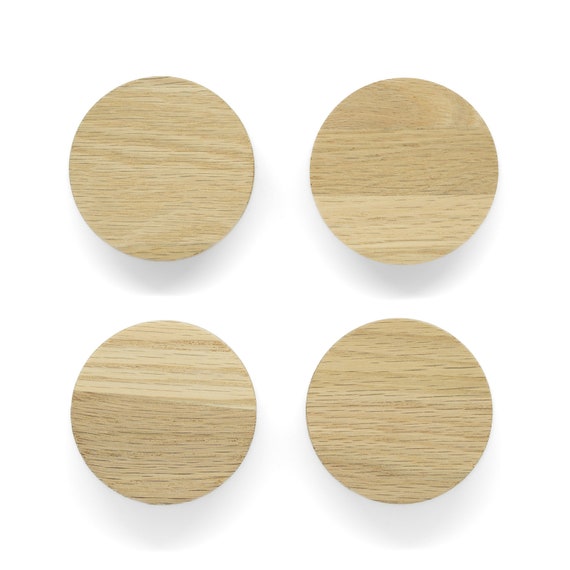The image is a detailed color photograph of four uniform, perfectly circular wooden coasters, arranged on a pristine white background. Each coaster showcases a unique wood grain pattern in light shades of beige, brown, and tan, emphasizing the natural variability of the material. These discs cast a subtle, gray shadow beneath them, creating a slight floating effect against the clean backdrop. The wood grain of each coaster is oriented horizontally, displaying bands of different hues arranged in a harmonious, organic fashion. The photograph is likely intended for online use, providing potential buyers with a clear and accurate representation of the coasters as a set, highlighting their craftsmanship and aesthetic appeal.